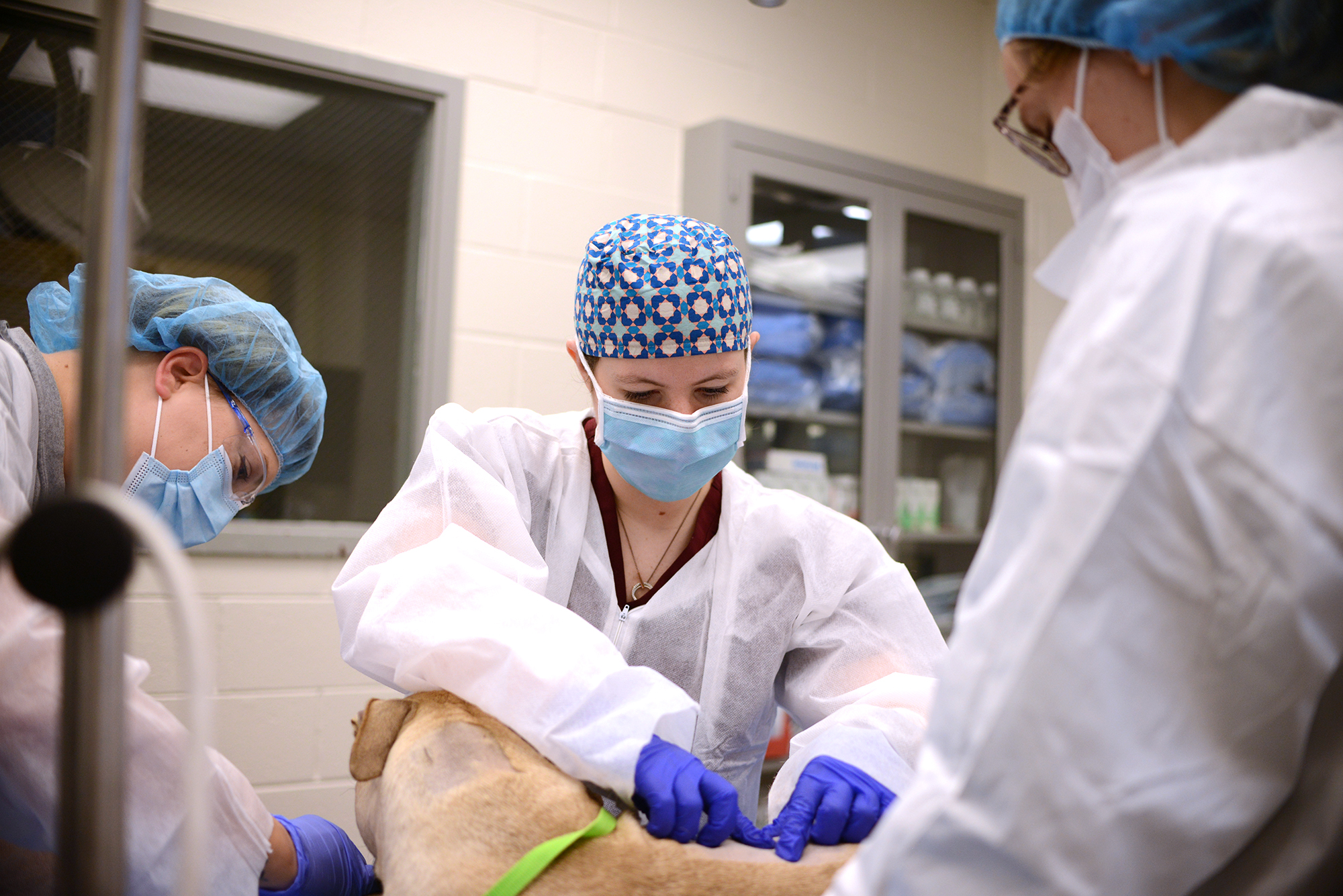In this detailed photograph, three female veterinarians are attentively working on a yellow Labrador in a concrete veterinary operating room. The room is equipped with a viewing window on the back wall, allowing observation from outside, and a gray metal cabinet with glass doors on the right, stocked with various medical supplies and equipment. Each veterinarian is dressed in a traditional white scrub, blue surgical masks, and latex gloves. They also all wear hairnets, with the middle veterinarian distinguishing herself by sporting a cloth bandana-style hairnet. 

The yellow Labrador has patches of fur shaved off around its neck and lower back, likely for the examination or treatment of wounds or possible surgical sites, as there are indications of a potential incision or scar behind its left ear. The dog is restrained with a bright green noose-style leash that secures it to the operating table. The veterinarian in the center, identifiable by her purple gloves and a distinctive necklace with a pendant, appears to be examining the shaved area on the dog’s back, while the other two stand on either side, potentially preparing or assisting in the procedure, though their specific actions are less clear. This seemingly routine yet meticulous procedure underlines the clinical and precise environment of the veterinary practice.